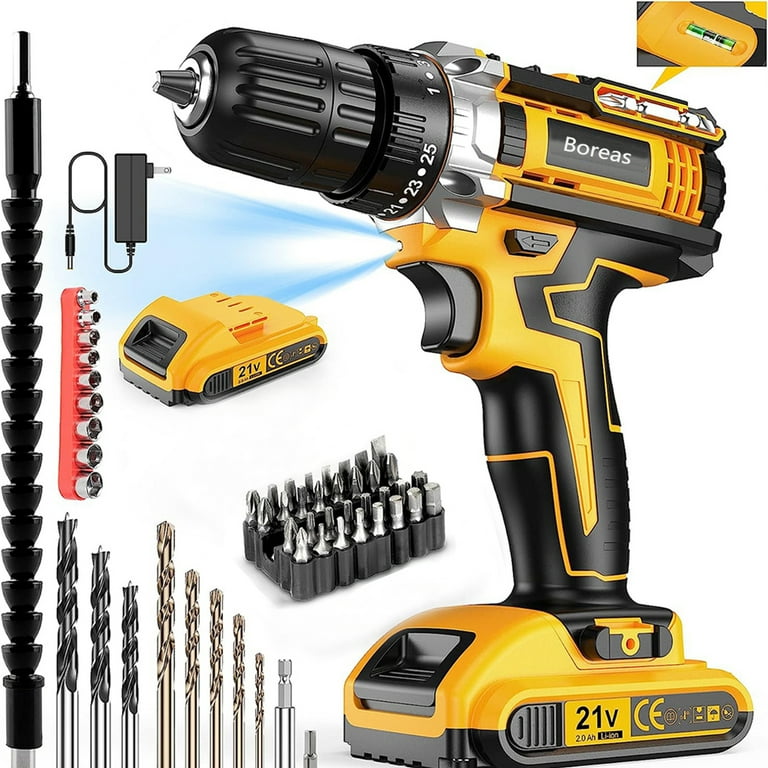This image features a striking yellow and black Boreas electric drill prominently displayed on the right side. The drill, which is battery-powered at 21 volts, is detailed with silver trim and bears the Boreas name in white letters. On the left side of the image, various components and accessories are neatly arranged. These include an assortment of drill bits, organized in a black container, an additional yellow and black battery pack, and an electrical charging cord. A distinct red container holds more specialized drill bits, while silver-toned drill bits are also visible. There is a long black attachment piece on the furthest left. Notably, the drill itself includes a blue light for precision and a built-in level for accurate alignment. The entire setup is set against a crisp white background, showcasing the organized and functional design of the drill and its accompanying parts.